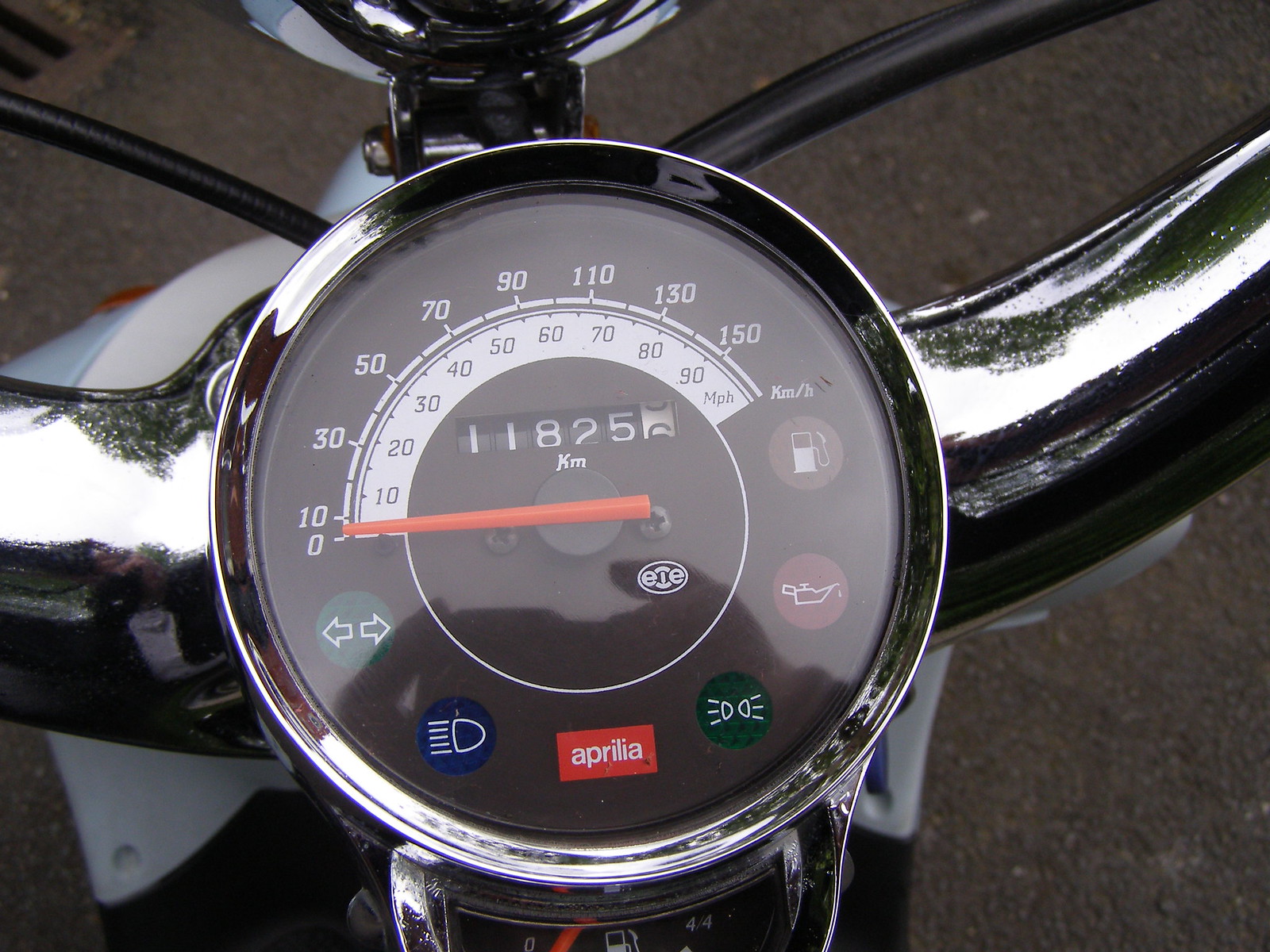The image captures a detailed view of an Aprilia motorbike's speedometer and odometer, with a predominant downward angle. The circular instrument cluster is silver-trimmed with a sleek black background. The speedometer displays measurements in both miles per hour, ranging up to 90 mph, and kilometers per hour, with a maximum of 150 kph. Currently, the speed needle rests at 0. 

The odometer reveals a total distance of 11,825.56 kilometers traveled. Surrounding the odometer, indicator lights for high beam, oil, and petrol are also visible, though none are illuminated at this moment. The word "Aprilia," denoting the bike's brand, is prominently displayed.

The silver-colored handlebars extend outwards, reflecting the sky, trees, and bushes in their polished surfaces. Below the handlebars, the bike's front section, including the headlight, can be partially seen, though the front wheel itself is out of view. The surrounding roadway, viewed from above, features a dark grey-brown asphalt surface. There is also a distinctive grate evident in the top left corner, adding texture to the road scene.